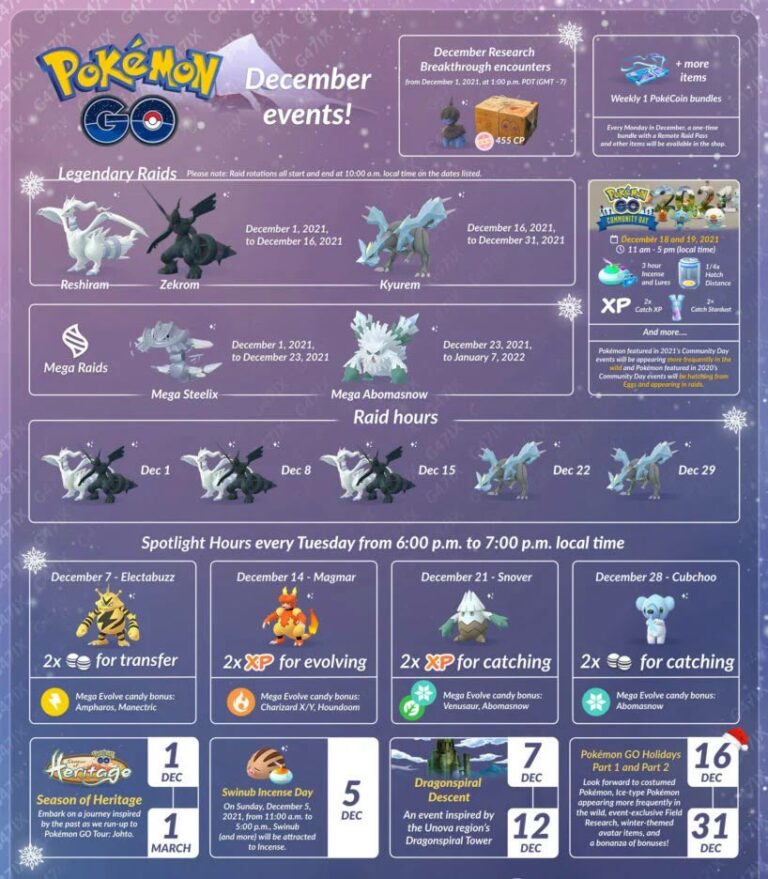This is a screenshot of what appears to be the official Pokémon Go website. The background features a gradient of purple, starting with a deep shade at the bottom and gradually lightening towards the top. A noticeable watermark reading "G47IX" spans the lighter section at the top of the page.

In the upper-left corner, the Pokémon Go logo is prominently displayed. The logo features the iconic yellow "Pokémon" text with "Go" underneath, rendered in blue and dark blue hues. A Poké Ball is cleverly embedded in the center of the 'O' in "Go." 

Adjacent to the logo, "December Events" is prominently listed, capturing the viewer’s attention. The main body of the page is dedicated to detailing several upcoming events:

1. **Season of Heritage**: December 1 - March 1
2. **Swinub Incense Day**: December 5
3. **Dragon Spiral Descent**: December 7 - December 12
4. **Pokémon Go Holidays, Part 1**: December 16 - December 31
5. **Pokémon Go Holidays, Part 2**: Same as above.

Scattered across the center and bottom sections of the webpage are various Pokémon characters, alongside additional event-related information and corresponding dates. This screenshot effectively captures the excitement and planning of December events for Pokémon Go enthusiasts.